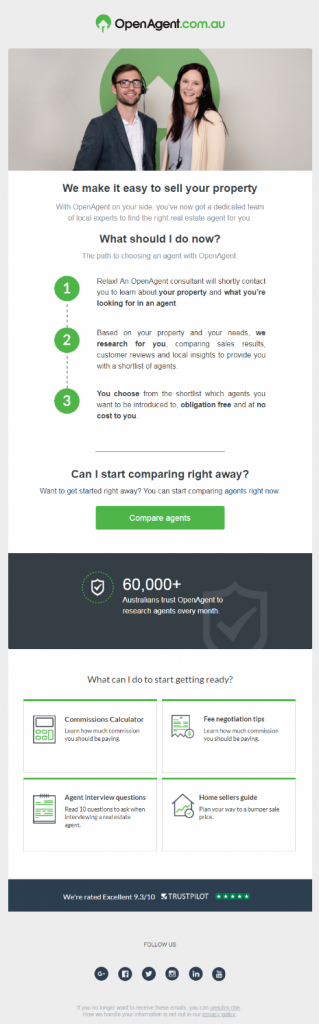In the photographic image, we see a web page interface. Dominating the top portion of the page, there's a circular green button featuring a white house graphic and black text that reads "Open Agent." The domain ".com.au" is also presented in green text. Prominently displayed at the top are two attractive individuals: a man with brown hair, glasses, and a headset, dressed in a suit coat and a button-down white shirt, smiling directly at the camera, and a woman with brown hair, a white cardigan, a blue shirt, and a headset, also smiling at the camera. They stand in front of a gray wall that features the same green logo bearing the white house and the slogan, "We make it easy to sell your property."

Just below this image, the text "With Open Agent on your side, you've now got a..." begins to trail off, making it difficult to decipher the rest. Below, there are three green buttons labeled "1," "2," and "3," accompanied by the question, "Can I start comparing right away?" To the right, a prominent green button reads "Compare now." 

A gray banner beneath these elements displays the text "60,000+" alongside a white shield icon. Finally, at the bottom of the page, social media icons for Facebook, Twitter, and Instagram are visible.